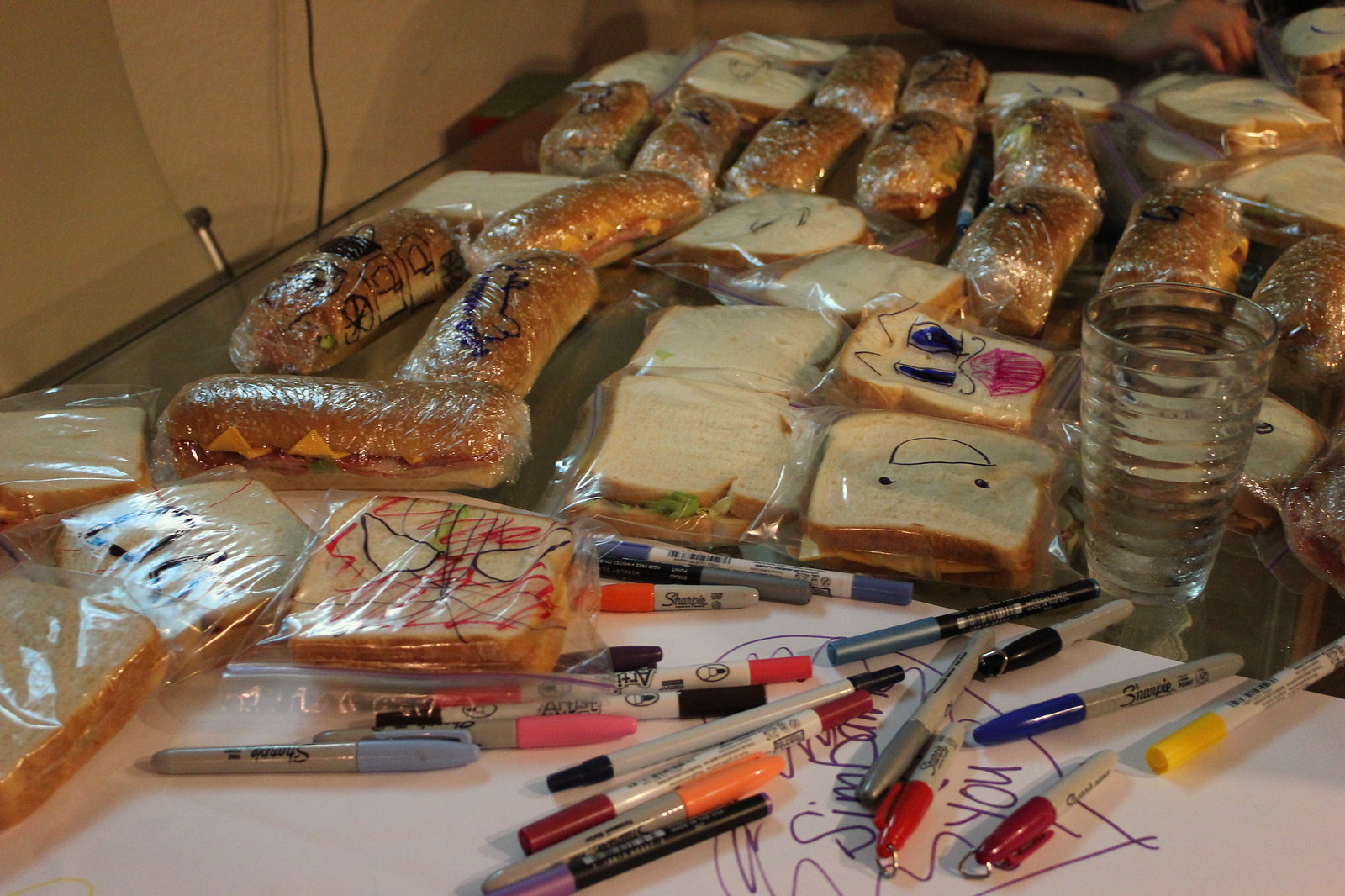In this detailed image, a variety of sandwiches are arranged on a metal table, all wrapped in either plastic wrap or plastic bags. The sandwiches come in different forms: some made with traditional white sandwich bread, while others are prepared with sub rolls, visibly containing ingredients like ham, cheese, and lettuce. Scattered among the sandwiches, a multitude of Sharpie markers in colors ranging from pale blue, pink, black, peach, maroon, yellow, dark blue, metallic blue, orange, and purple can be seen. Some of the plastic wrap on the sandwiches is decorated with faces and playful drawings, such as smiley faces and a possible cat illustration, indicating a touch of creative labeling, possibly by kids.

A cup, perhaps half-filled with water, designed with horizontal ribs, rests on the right side of the table. There's a piece of paper with a heart drawing, scribbles, and the words "Simba and You" written in purple ink. A person's hand is partially visible in the far corner, and a power cord can be spotted hanging against the stark white wall in the background, adding to the casual, laid-back atmosphere likely indicative of a lunch preparation or charity event.